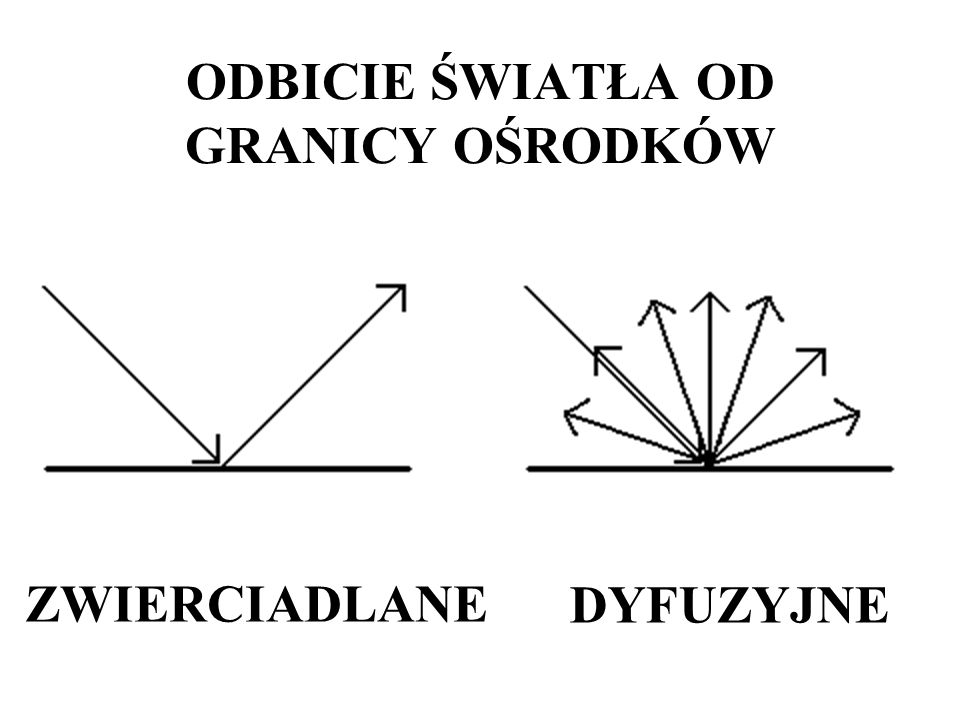The image is in black and white, featuring black text and two arrow diagrams on a white background. The text, likely in Polish, reads "Odbicie Światła od Granicy ośrodka" at the top, centered in bold, black letters. The first diagram, located on the left, includes a horizontal black line with one arrow descending diagonally from the upper left at a 45-degree angle towards the center, terminating at the line, and a second arrow ascending from this point at a 45-degree angle towards the upper right. Beneath this left diagram is the word "Zwierciadlane."

The second diagram, placed to the right of the first, also has a similar horizontal black line with a single arrow approaching the line at a 45-degree angle, but instead of just one arrow pointing upwards, it has seven arrows radiating upwards in a fan-like pattern. The arrows emerge from multiple points along the line, with one arrow pointing directly upwards and the others spreading out at various angles to the left and right. Below this right diagram is the word "Dyfuzyjne."